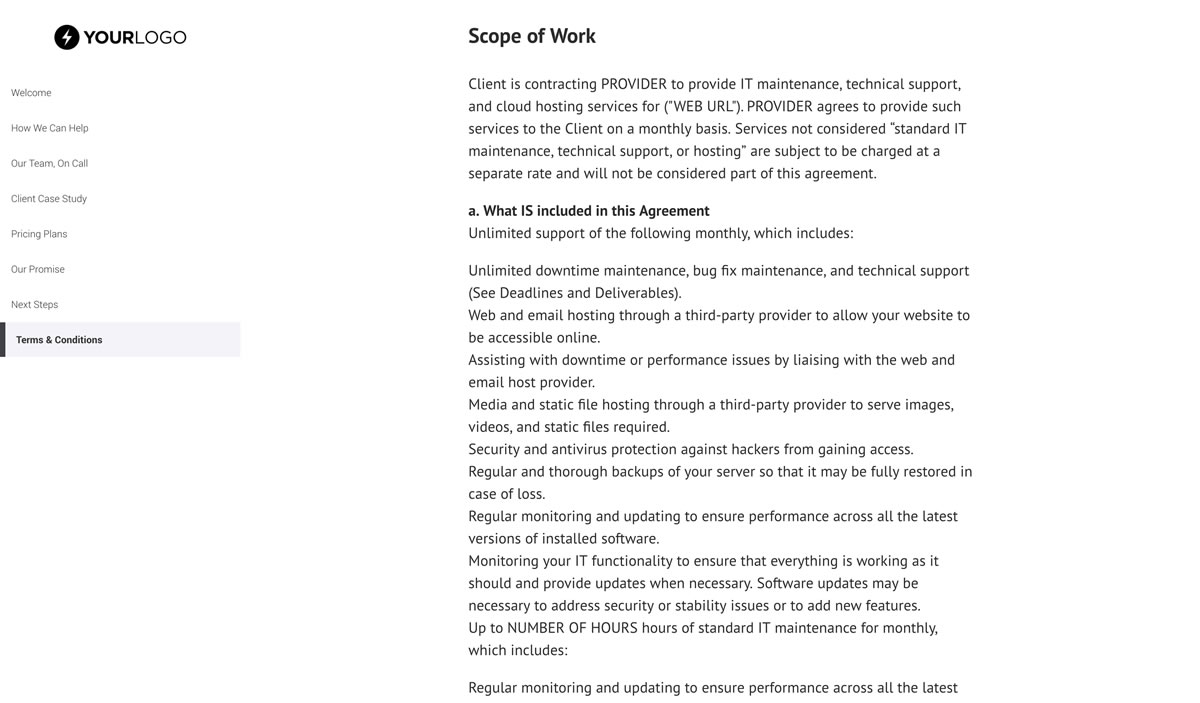**Caption:**

On a clean, white background, the left-hand side prominently features the title "Your Logo," with "Your" rendered in bold black and "Logo" in a lighter gray. Beneath this, in small gray letters, is a list of navigation options: "Welcome," "How We Can Help," "Our Team on Call," "Client Case Study," "Pricing Plans," "Our Promise," and "Next Steps." Further down, a gray banner spans the width of the page, with the text "Terms and Conditions" in stark black letters.

Centered on the page, "Scope of Work" is displayed in bold black. Below this title, in gray text, the document details: "The client is contracting the provider to offer IT maintenance, technical support, and cloud hosting services for a specified web URL. The provider agrees to render these services on a monthly basis. Any services beyond standard IT maintenance, technical support, or hosting will incur additional charges and are not included in this agreement."

Following this are more detailed sections:

**Clause A: What's Included in This Agreement?**

In this section, gray text elaborates:
- Unlimited monthly support covering:
  - Downtime management
  - Maintenance and bug fixes
  - Adherence to set deadlines and deliverables
  - Web and email hosting through a third-party provider ensuring website accessibility
  - Assistance with downtime or performance issues by coordinating with the web and email host provider
  - Media and static file hosting via a third-party provider for images, videos, and static files
  - Security and antivirus measures to prevent unauthorized access
  - Regular, comprehensive server backups for full restoration if needed
  - Continuous monitoring and updates to maintain performance with the latest software versions
  - Monitoring IT functionality to ensure optimal operation, providing updates as necessary. This includes software updates for security, stability, or new features.
  
Additionally, the agreement includes up to a specified number of monthly hours dedicated to standard IT maintenance tasks such as ongoing system monitoring and updates, although this section is cut off and incomplete.